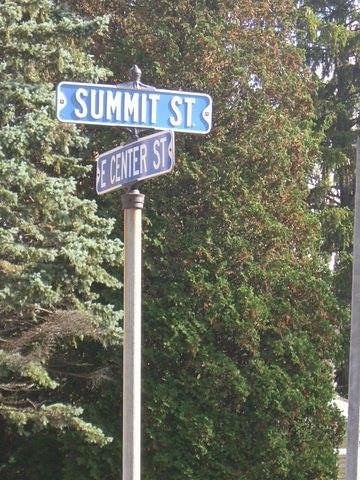In this vibrant outdoor photograph, we observe a bright daylight setting that accentuates the natural greenery encompassing the area. The image prominently features several trees in the background, their foliage a mix of rich green and lighter green hues, adding depth and vitality to the scenery. These trees, which could either be quite large or simply appear so due to the photograph's close-up perspective, create a lush backdrop. In the foreground stands a street sign mounted on a sleek white support pole. The sign comprises two long, rectangular markers, each facing opposite directions. Both signs are distinct with their white text on blue backgrounds, with the top sign reading "Summit Street" and the bottom sign indicating "East Center Street." This detailed description captures the serene yet structured essence of the photograph, blending natural and urban elements.